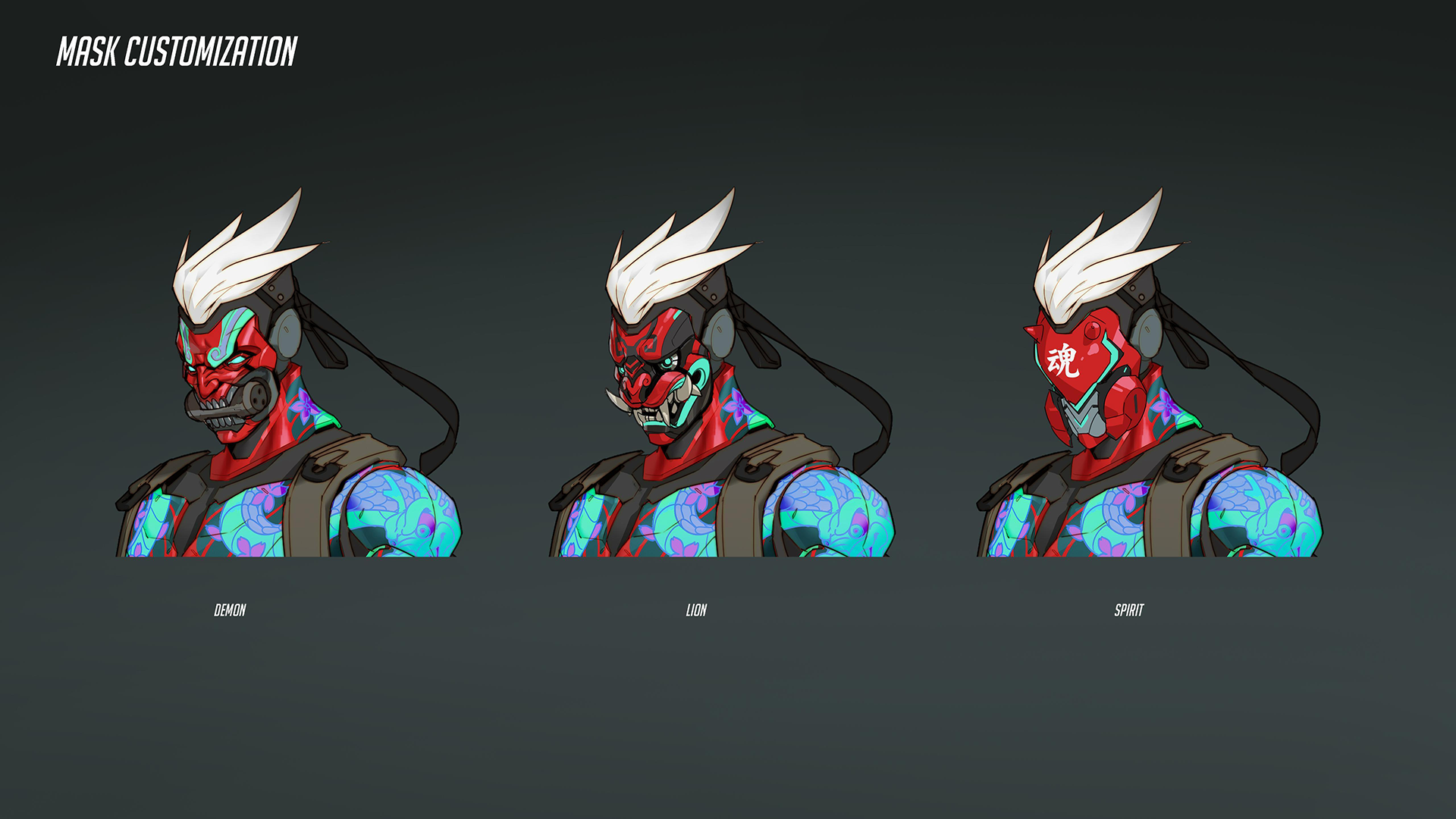Set against a dark gray or blackish backdrop, the image features the text "MASK CUSTOMIZATION" in bold white capital letters in the top left corner. Centered across the image are three similar gaming characters depicted from the shoulders up, each with a distinct red face and neck, slicked-back white hair with black coverings over the back of their heads and ears, and a ribbon extending towards their left shoulder. They are all sporting bright green, blue, and purple chests adorned with a floral design and wearing straps over both shoulders. Each character's mask and details vary significantly:

1. The first character, labeled "DEMON" in white text beneath, has teal eyebrows, blue swirls near the bridge of the nose, and a contraption held in its mouth akin to a dog biting a bone.

2. The second character, labeled "LION," features a snarling lion mask with sharp white teeth and teal accents around the lips.

3. The third character, labeled "SPIRIT," has a more abstract mask with a thin teal line for eyes, a gray shield-like cover over the mouth, and red cylinders resembling gas mask filters on either side. 

All three characters gaze towards the left side of the image, unified by their differing yet strikingly detailed masks.